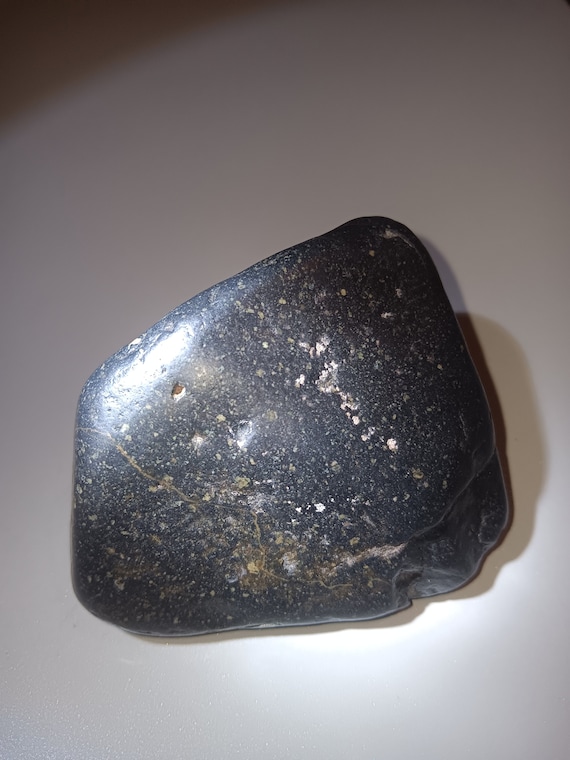The image depicts a small, lightweight black stone positioned against a clean white background, possibly on a surface like a table. The stone draws the eye with its smooth yet worn appearance, featuring various nicks, spots, and a mixture of white and brown markings indicative of age and use. Particularly noticeable are the white crystal-like nicks scattered across its surface and an orangey-brown rust-like patch toward the middle bottom. The stone is roughly rectangular, albeit with a slightly distorted shape, and has a prominent shine on its upper left that casts a shadow to the right. The highlighted, bright spot on the upper left adds a reflective glare, further emphasizing its polished yet rugged texture. Overall, this stone appears as if it might be found at the bottom of a planter, adding a naturalistic, rustic charm to its surroundings.